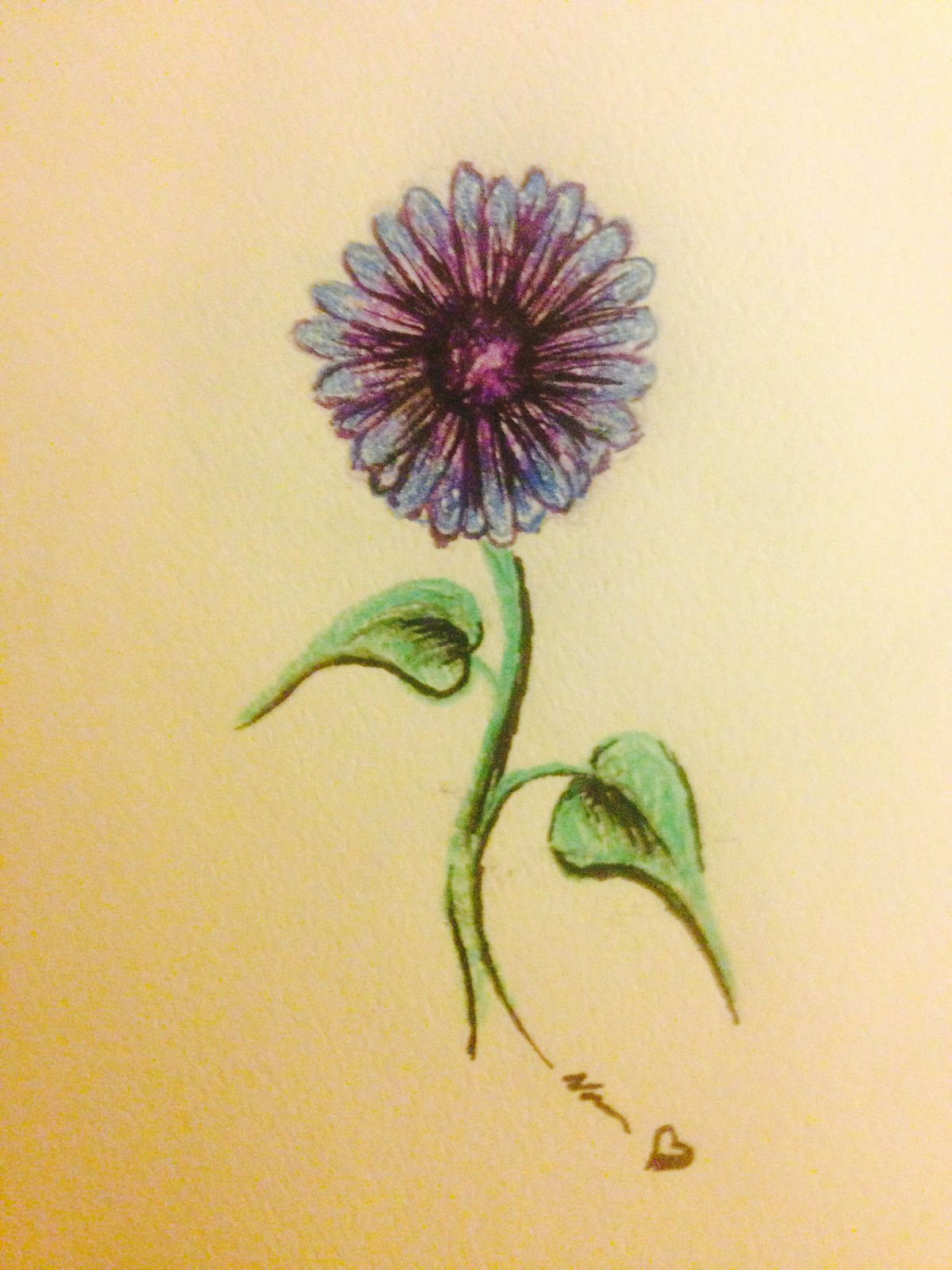This photograph captures a detailed drawing of a flower on a yellowish-tan piece of paper. The flower, situated in the center about two inches from the top, features a cluster of multicolored petals that are flat yet rounded at the ends. The petals exhibit gradations from gray-green on the outer edges transitioning through pinks and oranges, culminating in a deep purple center with yellow and pink highlights. The flower’s core is dark purple, encircled by black, and the tips show hints of white. Below the bloom, a thin green stem, shaped like a backward S-curve, descends. Two green leaves, each shadowed to indicate a bend, sprout from the stem at different levels and angles, both gently drooping downwards. At the bottom right of the stem, the artist has signed their name, which appears to be "Norm" or "Norma," in brown ink, accompanied by a small brown heart. The overall lighting of the photograph is slightly brighter on the right side, suggesting a peachy background possibly due to an external light source.